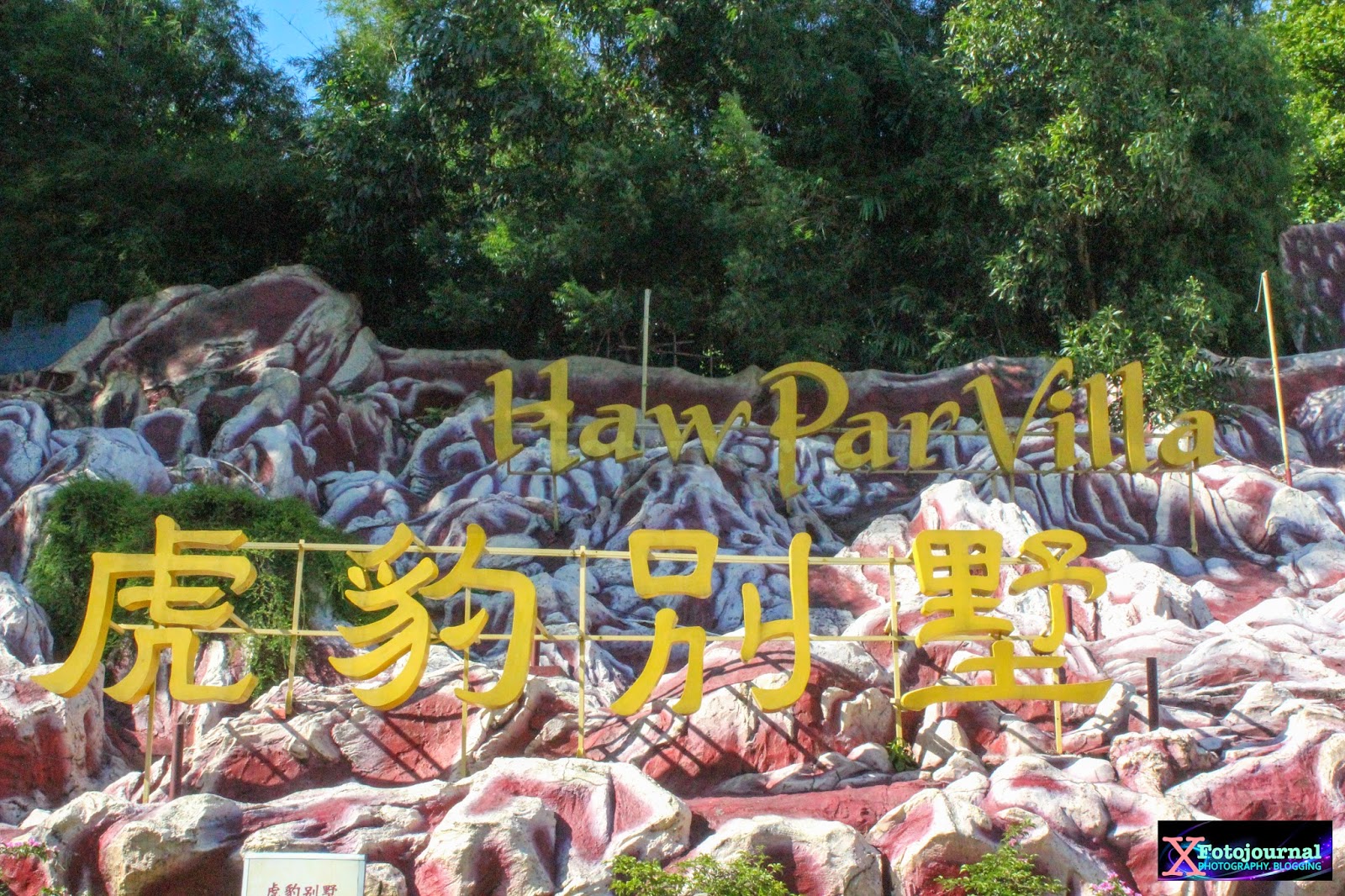This outdoor photograph features a faux rock formation painted in pinkish-red hues with white outlines, giving it a styrofoam-like appearance. Mounted on the rock formation, a yellow sign reads "HAW PAR VILLA" with Mandarin characters below it. Another yellow Mandarin sign is positioned to the left, and there's a small white information sign with more Mandarin characters at the bottom left. Green trees frame the top of the image, allowing a glimpse of blue sky through their leaves. A leafy green bush is visible on the left side of the rock formation, and a bit of grass or bushes can be seen at the very bottom. The image is credited to a "PHOTO JOURNAL," indicated by a logo in the bottom right corner, featuring a purple swirl and the text "FOTO Journal."